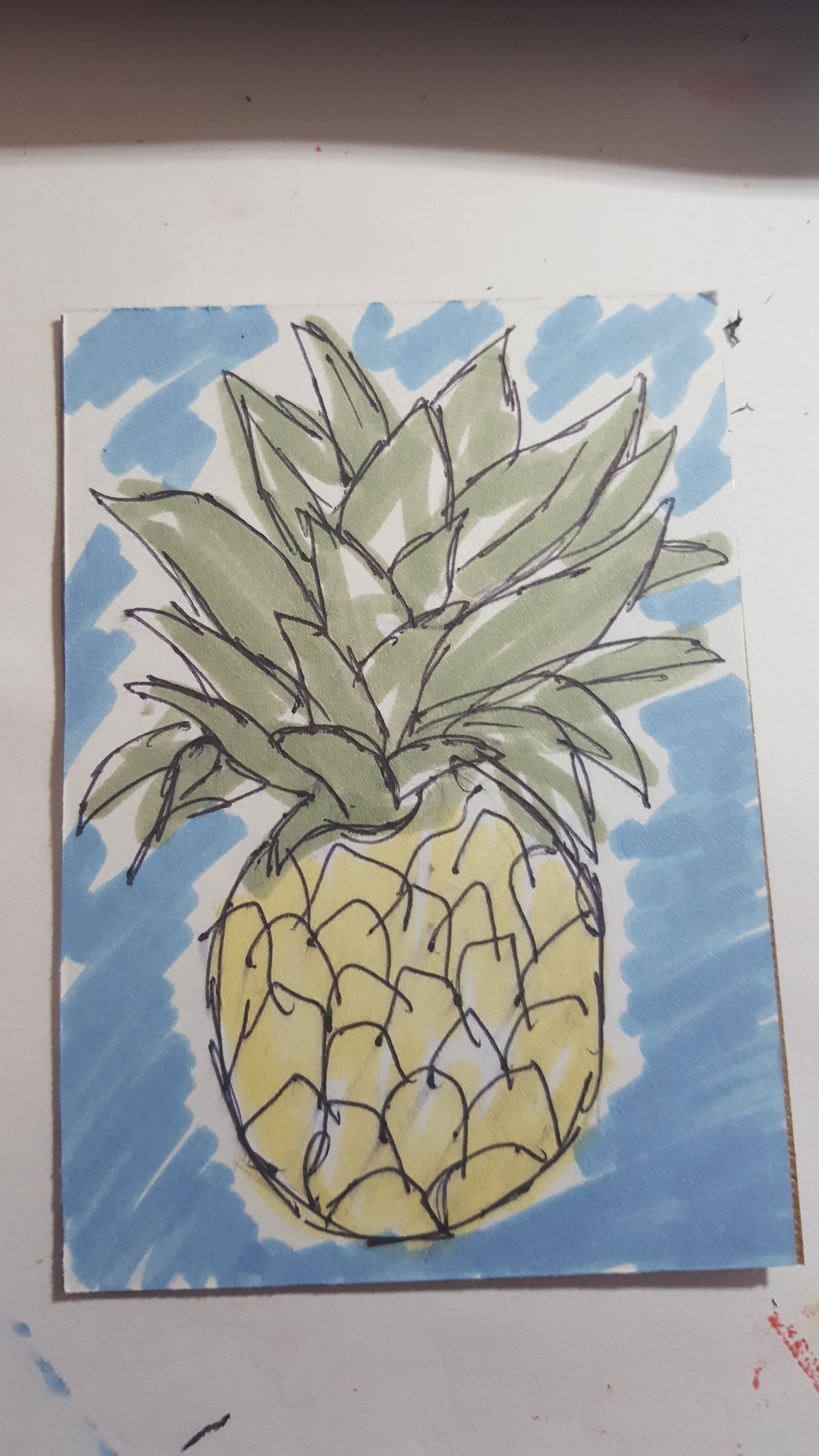The image displays a detailed drawing of a pineapple on a small canvas, situated on a white surface. The background features a horizontally shaded light blue color with some white areas peeking through. The pineapple itself stands prominently, outlined in black. The base of the pineapple is colored yellow, accentuated with black lines to indicate its scaly texture. The top of the pineapple showcases a full head of spiky green leaves, also outlined in black, with various leaf patterns bending upwards and downwards. This artistic piece, likely created using felt-tip pens or vivid colored pencils, conveys a simple yet instantly recognizable representation of a pineapple. Despite a quick coloring process, the drawing exhibits a lively and charming portrayal. There are also some minor red and green marks on the white surface surrounding the canvas.